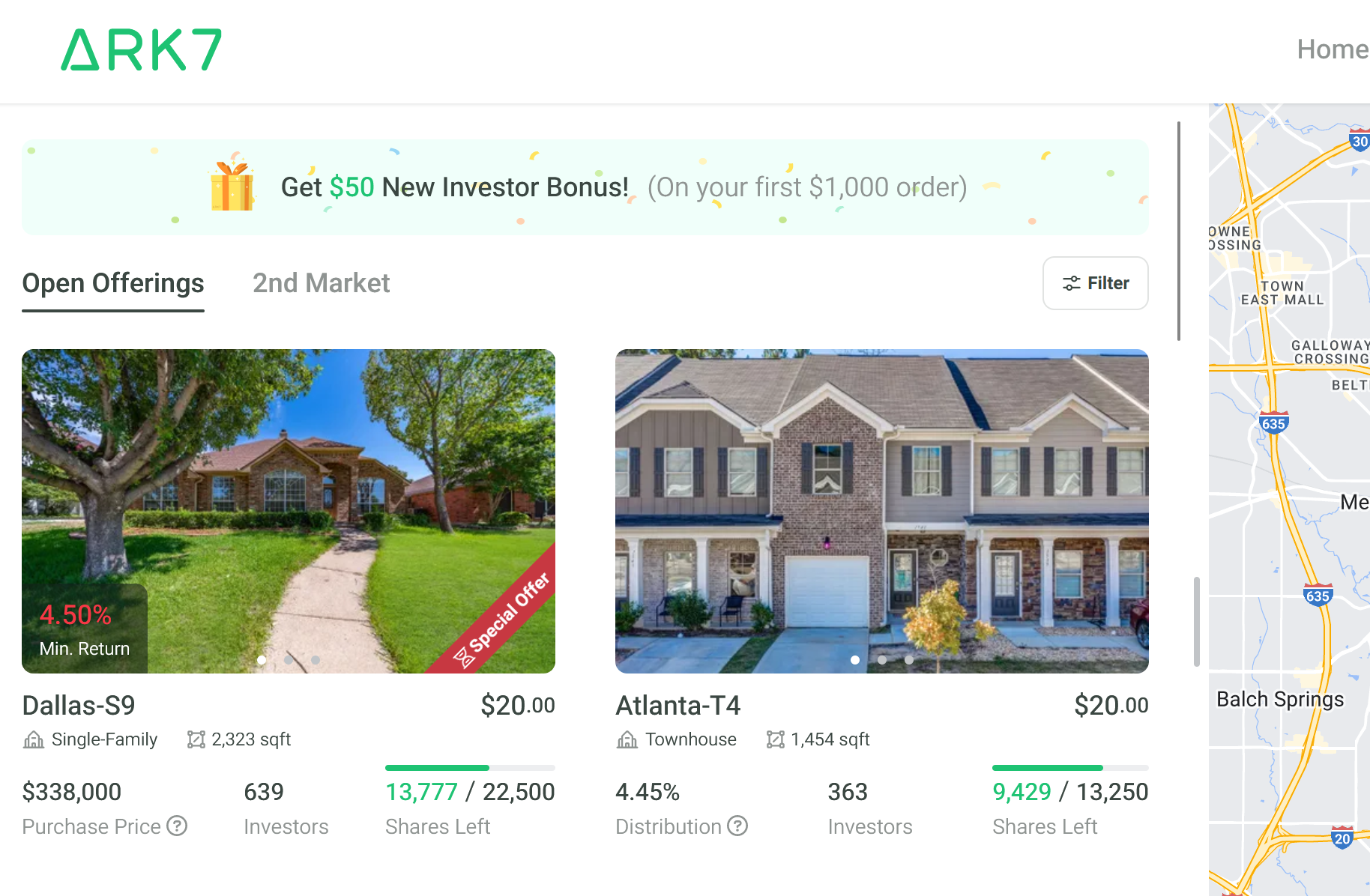On the website, prominently displayed in the upper left corner, a stylized green triangle resembling an 'A' and marked with 'RK7' sits against a white backdrop. To the right, a gray 'Home' icon introduces the top navigation. Directly below this top section is a dividing line, under which a colorful banner catches the eye. The banner, predominantly green, showcases a yellow and orange package with text promoting a bonus: "Get $50 New Investor Bonus on Your First $1,000 Order."

Beneath this promotional banner, the website details various sections, notably "Open Offerings" and "Second Market". The main content area features images of two different properties along with a map displayed on the right side. 

The first property, labeled 'Dallas S9', is a single-family home boasting 2,323 square feet. It's listed as a special offer requiring $20 for a 4.50% minimum return. The purchase price for this property is $338,000, and it has already attracted 638 investors. There remain 13,777 of the initial 22,500 shares available for investment, indicating an opportunity to buy equity in this house.

The second property, 'Atlanta T4', is a townhouse with a size of 1,454 square feet. The investment terms are similar, with a $20 minimum and an anticipated 4.45% return distribution. 

This detailed layout and structured information on the site guide potential investors through the process of buying shares in real estate properties, illustrating the platform's offerings and incentives clearly.